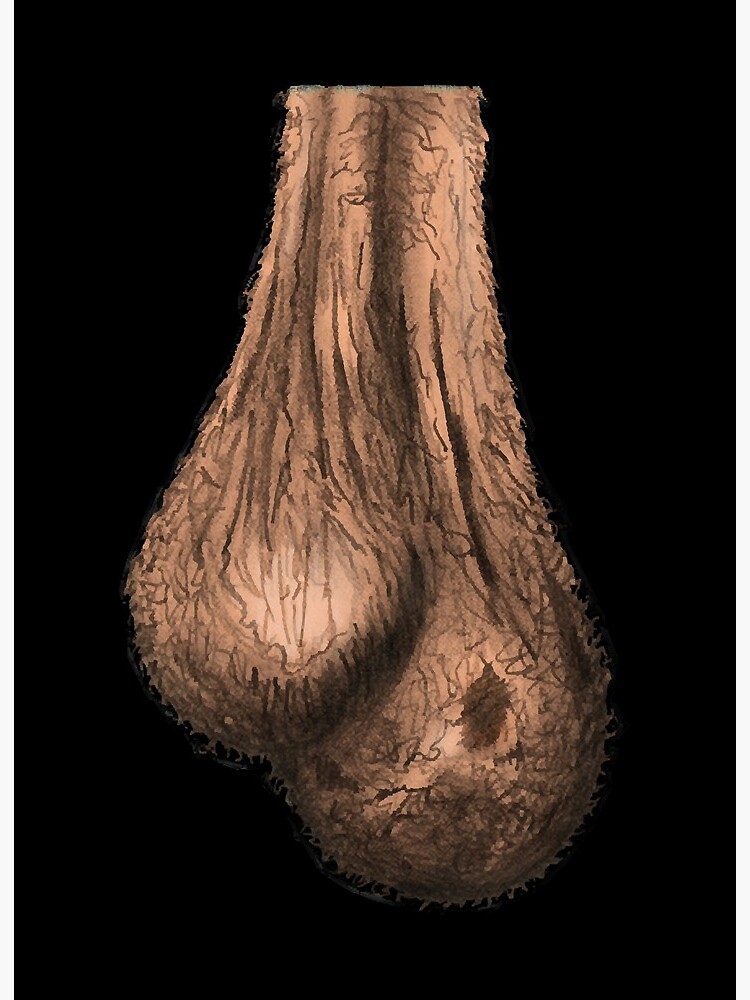The image is a highly detailed and realistic digital illustration of a man's testicles, set against a completely black background. The testicles are depicted with notable texture, including wrinkled, stretched-out skin and intricate shading that gives them a lifelike appearance. The left testicle hangs slightly higher than the right, with beige skin accented by brown shading, particularly around the bottom. The illustration includes numerous squiggly lines representing pubic hair, adding to its realistic detail. There is also a prominent brown spot on the center of the right testicle, possibly intended to depict shadow. The overall artwork showcases an impressive use of light and shadow, making it appear quite realistic despite its crude subject matter.